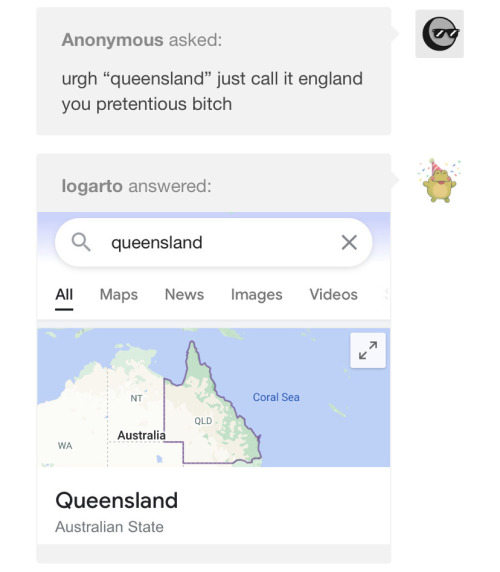The image is a screenshot of two text messages. 

The first message is from an anonymous user, represented by an icon of a circle with sunglasses. The text reads, "Anonymous asked: 'U-R-G-H, Queensland, just call it England, you pretentious bitch.'"

The second message is from a user with an avatar of a small tan-colored animated hippo wearing a party hat. The text is from a user named "LOGARTO" and reads: "LOGARTO answered." It features a search bar displaying the word "Queensland," with options for "All," "Maps," "News," "Images," and "Videos" beneath it; "All" is highlighted. The image below the text shows a map of Australia, highlighting the region of Queensland to the right, with the Coral Sea adjacent to it. Neighboring areas labeled "NT" (Northern Territory) and "WA" (Western Australia) are visible. Underneath the highlighted area, the label reads "Queensland," with a subtitle stating "Australian state."